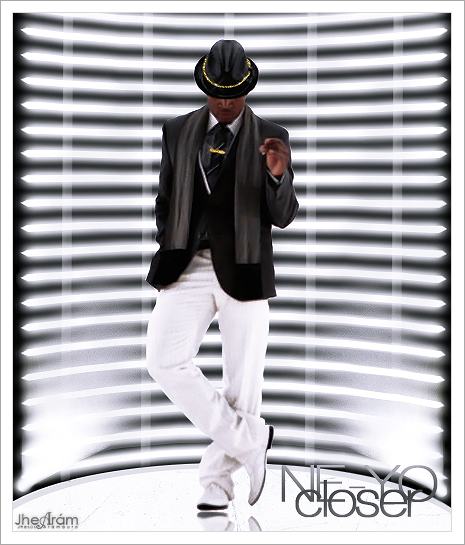The image appears to be an album cover or poster of the artist Ne-Yo, prominently labeled "Ne-Yo Closer" in the bottom right corner. Ne-Yo, dressed in a sophisticated and stylish ensemble, is striking a pose while looking downward, revealing only his nose and chin. His attire includes a black fedora with a gold rim, a black jacket over a white collared shirt, and a grey scarf draped around his neck, possibly accessorized with a gold tie or tie clip. He also sports white pants and matching white shoes, exuding a sharp, monochromatic look. Ne-Yo stands on a white podium, against a dramatic backdrop: white horizontal blinds curve around him, contrasting with the black background, and the floor beneath him is illuminated to enhance the visual impact.